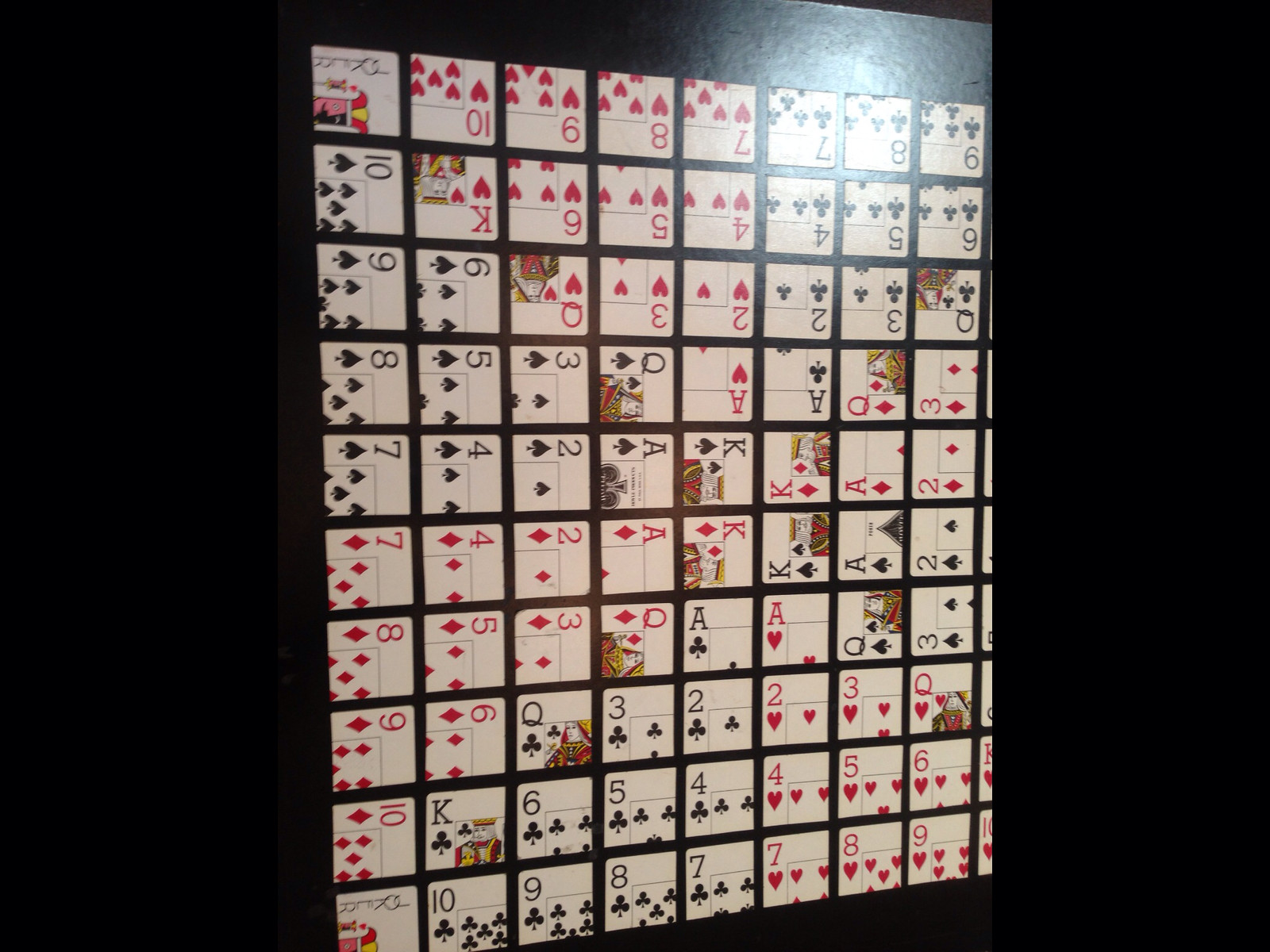The image showcases a striking display of playing cards meticulously arranged in a grid formation on a jet black wall. The black backdrop is consistent across the far left, right, and above the cards, which adds a stark contrast to their white backgrounds, creating a dramatic visual effect. 

The playing cards are divided both horizontally and vertically by thin black strips, giving the installation a sense of order and structure. A soft light illuminates the cards and the upper part of the wall, emphasizing their details. 

Starting from the upper left, a Joker card is prominently positioned. As we move through the columns from left to right, we come across a sequence of cards that in some cases, are only partially visible or presented at various angles, adding an intricate touch to the arrangement. 

In the next sequence, we can identify cards such as the ten, nine, eight, and seven of hearts, alongside the seven, eight, and nine of clubs. Below the Joker on the far left, an array of cards including the ten of spades and king of hearts are discernible, following the order of six, five, and four of hearts, and four, five, and six of clubs.

Moving further to the right, the cards include the nine and six of spades, and an upside-down queen of hearts among others. This upside-down queen is part of a broader pattern where many cards are oriented inversely, save for those on the far left which are angled upright.

The third column reveals cards like the eight of spades, five of spades, and three of spades, with the queen of spades oriented correctly on their side. Following this, the ace of hearts and ace of clubs are upside down, while the queen and three of diamonds face the opposite direction. 

Continuing, we see the seven, four, two, and ace of spades arranged in order, followed by the king of spades and ace of diamonds facing to the right. As the sequence continues, it becomes evident that cards like the king and ace of diamonds, two of diamonds, seven of diamonds, and more proceed until breaking into a varying orientation yet again.

Towards the final segments, the sequence includes the ten of diamonds facing upright, the king of clubs, and cards like the six, five, and four of clubs, interspersed with hearts. Pertinent to the arrangement, the final columns depict sequences that range from more predominate clubs to intermixing with heart suits, concluding with another joker card.

The overall effect is a captivating display that merges the disciplined arrangement of cards with the intriguing interplay of orientations and light, generating a sense of ordered chaos.